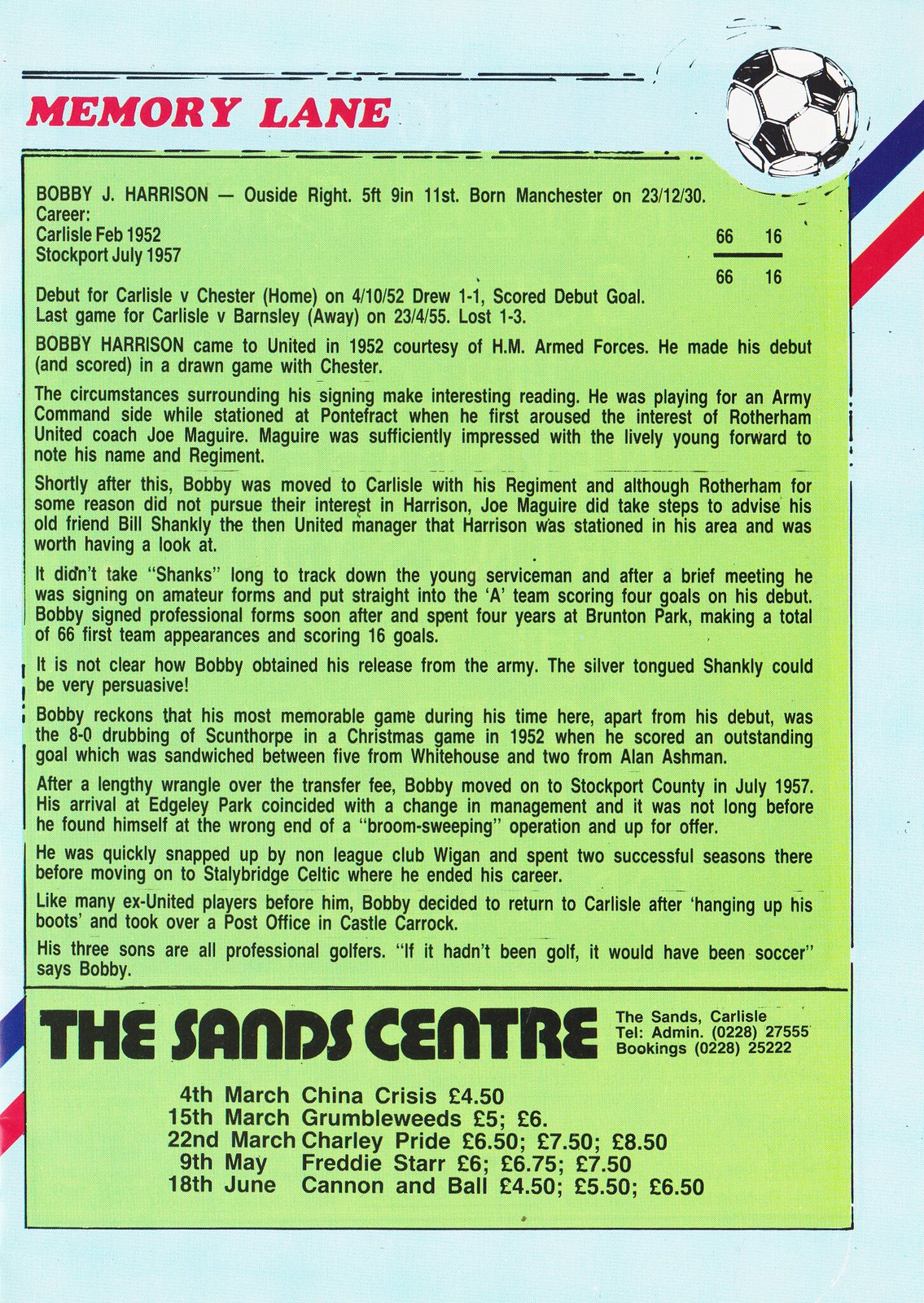This vibrant page from a sports program, titled "Memory Lane," captures the remarkable journey of soccer player Bobby R. Harrison. The photograph of the printed page features a header with the title "Memory Lane" in bold red letters and a graphic of a soccer ball in the top right corner. 

The central focus is a green box with black print detailing Bobby's profile and career milestones: "Bobby R. Harrison, outside right, 5 feet 9 inches, 11 stone, born Manchester on 23 December 1930." It outlines his career trajectory from Carlisle in February 1952 to Stockport in July 1957. Key highlights include his debut for Carlisle against Chester on 4 October 1952, where he scored in a 1-1 draw, and his last game for Carlisle against Barnsley on 23 April 1955, ending in a 1-3 loss.

Bobby joined United in 1952 via HM Armed Forces and quickly impressed with his debut performance. His early talent piqued the interest of Rottingham United coach Joe Maguire, which led to a recommendation to United manager Bill Shankly. Harrison swiftly transitioned to professional status, making 66 first-team appearances and scoring 16 goals at Brenton Park within four years. Notable achievements include a standout game in 1952, where he contributed to an 8-0 victory over Southdorf with his stellar goal.

Later, Bobby's career saw him transition to Stockport County in 1957, followed by successful stints at non-league Wigan and Stanley Bridge Celtic, concluding his playing days. Post-retirement, he returned to Carlisle and ran a post office in Castle Carrick, while his three sons pursued careers as professional golfers.

The bottom of the page lists events at the Sands Center, Carlisle, with contact details: ADMIN 0228-2755 and bookings at 0228-2522. Upcoming events include performances by China Crisis on 14 March, Grumble Weeds on 15 March, Charlie Pride on 22 March, Freddie Starr on 9 May, and Cannon and Ball on 18 June. The page is accentuated by a diagonal blue and red stripe behind the green box, adding a dynamic visual element to the detailed recount of Bobby Harrison's storied career.